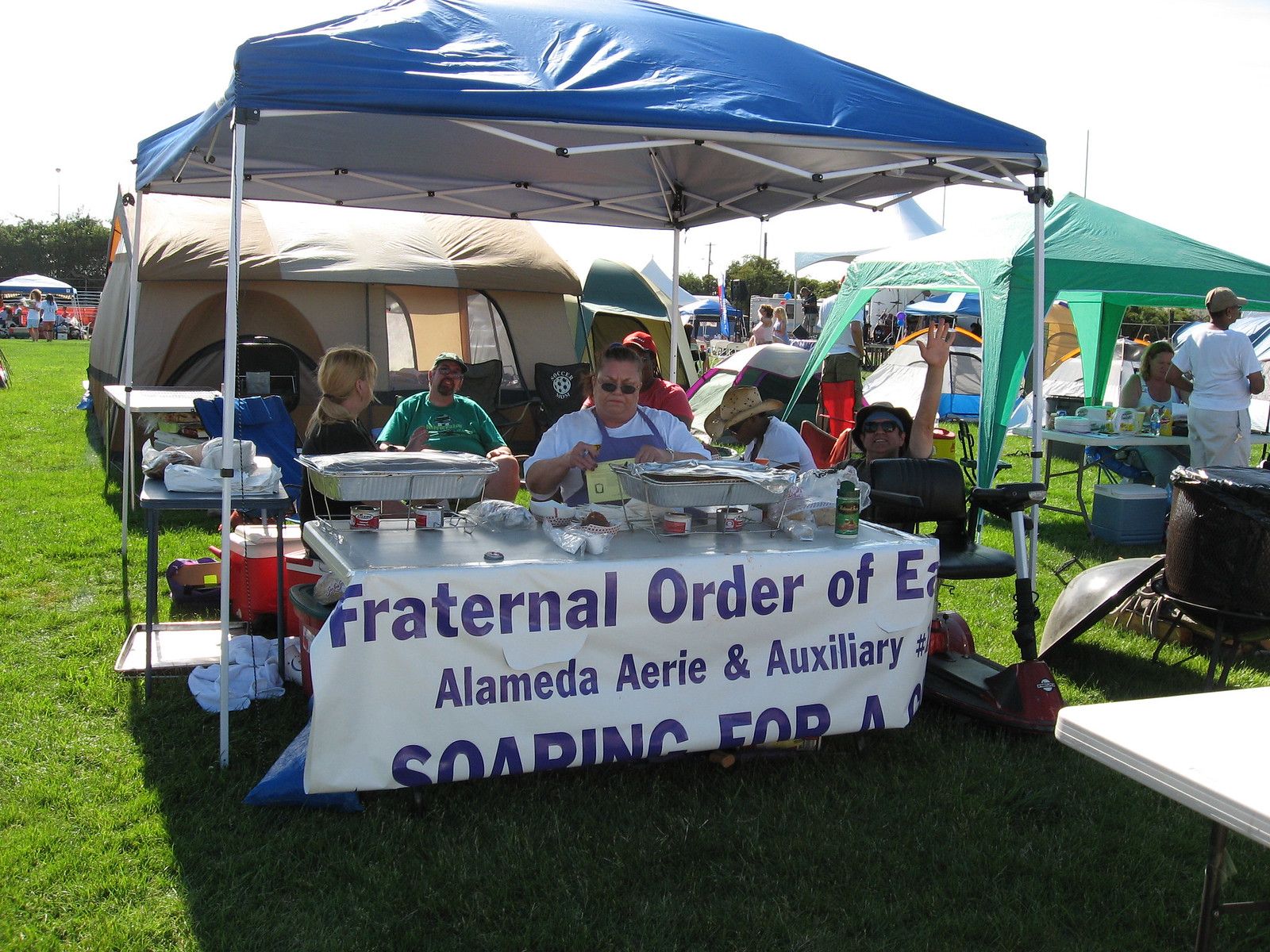This image depicts a vibrant outdoor fair taking place on a sunny day, with the setting adorned by a canopy of various shades including blue, green, and white. In the center, there is a blue pop-up tent sheltering a table draped with a white sign partially obscured and wrapped around the table edge, making some of the text unreadable. From the visible parts, the sign reads "Fraternal Order of Alameda Area and Auxiliary," embellished in dark blue or purple lettering. The table is topped with heating utensils and trays, suggesting food preparation or warming, with people seated around the table possibly engaging in culinary demonstrations or selling food items. The people in the scene are scattered on the green grassy surface beneath a sunny sky. A person wearing a purple apron is visibly involved in the activities behind the table. Surrounding this main booth are additional canopied tables, indicating bustling activity and an assortment of goods likely being sold or displayed. The overall atmosphere is lively, reflecting a community gathering such as a craft show or an outdoor farm fair, with a backdrop of trees and a portion of the sky visible, highlighting the mid-day ambiance.